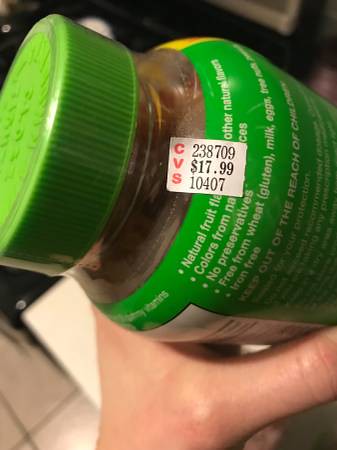This photograph captures a hand holding a clear plastic bottle from an overhead angle. Emerging from the center is the hand, with the thumb and thumb knuckle clearly visible, while the rest of the hand is obscured by the bottle. The bottle features a bright lime green cap wrapped in plastic film. Its neck is transparent, showcasing a green label with white lettering that runs along the side of the bottle. The bottle is tilted, providing a partial view of both its clear neck and the green-label section. A distinctive white square is positioned on the green label. Inside the square, to the left, the letters "CVS" are arranged vertically. On the right side of the square, three rows of black numbers are printed at the top.